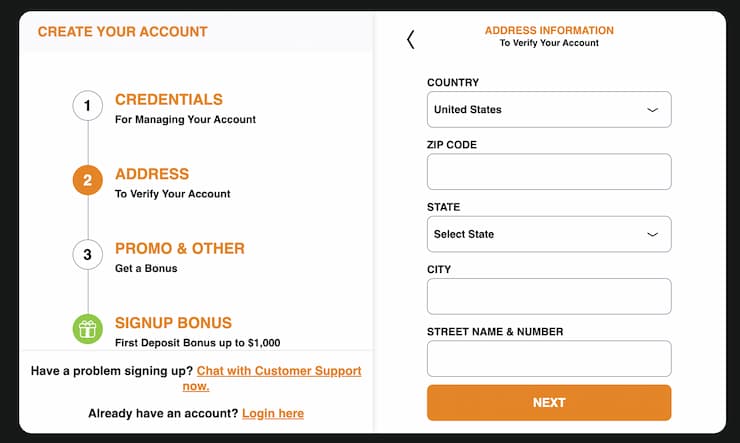The image showcases a web page with a black background behind the active window. The active web page features a predominantly white background accented by orange details. 

In the top left corner, the phrase "Create Your Account" is prominently displayed in orange font. Below this header, the account creation process is divided into three distinct steps:

1. **Credentials**: This section begins with a white bubble containing the black number "1." It is labeled "For managing your account" in black font.
  
2. **Address**: The second step is denoted by an orange button labeled "Address" with the number "2" highlighted in orange. The accompanying instruction, "To verify your account," is written in black font.
   
3. **Promo and Other**: This final step features a white bubble with the black number "3." The words "Promo and Other" are written in orange, and beneath it, "Get a bonus" is displayed in black font.

Further down, there's a green and white gift box with the text "Sign Up Bonus" in orange. Next to it, the benefit of a "First Deposit Bonus Up to $1000" is noted.

Near the bottom, a black font message reads, "Having a problem signing up?" followed by an orange button prompting users to "Chat with Customer Support Now." Lastly, for existing users, there is an orange font link stating, "Already have an account? Login here."